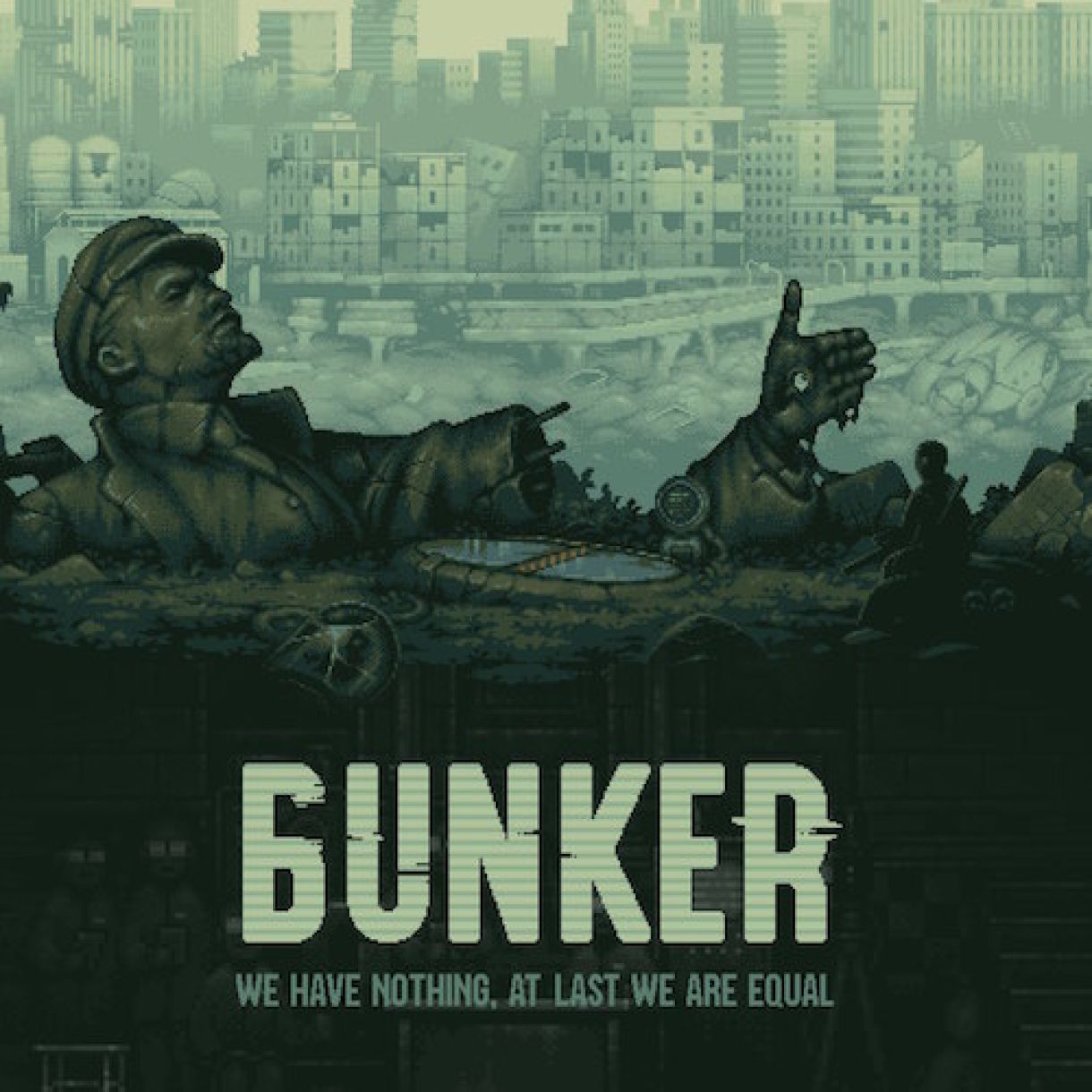In this detailed and evocative image, a pixelated cityscape unfolds, reminiscent of a modern hyper-realistic pixel game set in an apocalyptic world. The background is dominated by decaying city buildings in pale green and gray hues, with a collapsed road leading into a river churning with foamy water, littered with debris. On a hill stands the central focus: a weathered statue of a soldier, evocative of World War I. The statue, capped with a newspaper boy hat, holds up a bullet-riddled hand, a necklace draped over it. His left arm is severed at the elbow, appearing to transition into a mechanical form. This desolate scene is framed by a large, staticky block of text at the bottom, declaring in pale green letters, “BUNKER,” followed by the haunting phrase, “We have nothing, at last we are equal.” Below the statue, embedded in the rubble, is an entrance to a bunker, more pristine and inhabited by scientists, a stark contrast to the devastation above. As a whole, the image conveys a powerful narrative of equality born from shared desolation amidst the ruins of civilization.